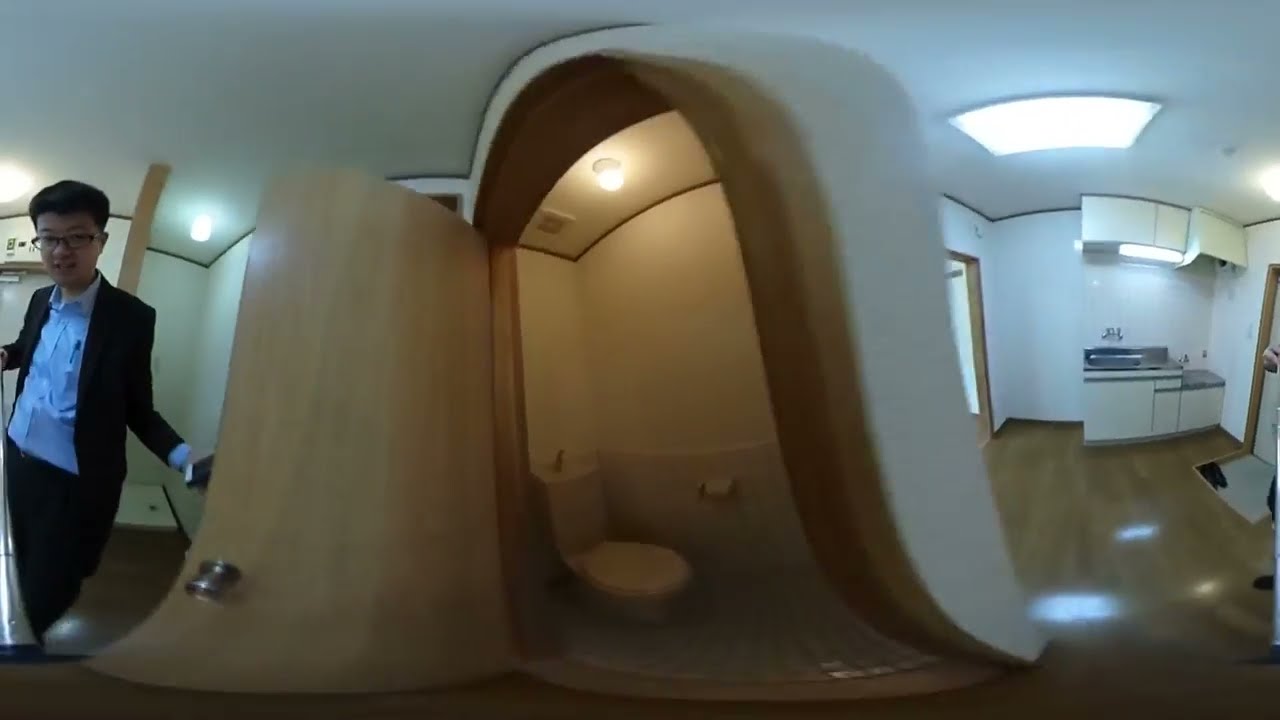The photograph showcases a panoramic view of an Asian apartment's interior, captured with a mildly distorted lens that wraps the scene into a circular vision. The image is framed by white walls adorned with wood-like colors, and wooden framed doors. On the far left, an Asian man dressed in a dark blazer, light blue shirt, slacks, black shoes, and glasses stands near a kitchenette, holding an indistinguishable object in his left hand. The kitchenette features a sink, countertop, tiled wall, hood, and bright fluorescent light. To the right of the man, a door with electronic equipment above it leads into the main living space. Further to the right, a cabinet and another doorway potentially leading to a bathroom are visible, along with a shiny brown floor. The far right of the image reveals a room in the background separated by a Japanese-style sliding door with a 2x5 grid of frosted windows. The scene is well-lit by multiple ceiling fluorescent lights, creating a bright, detailed view of the apartment's interior.